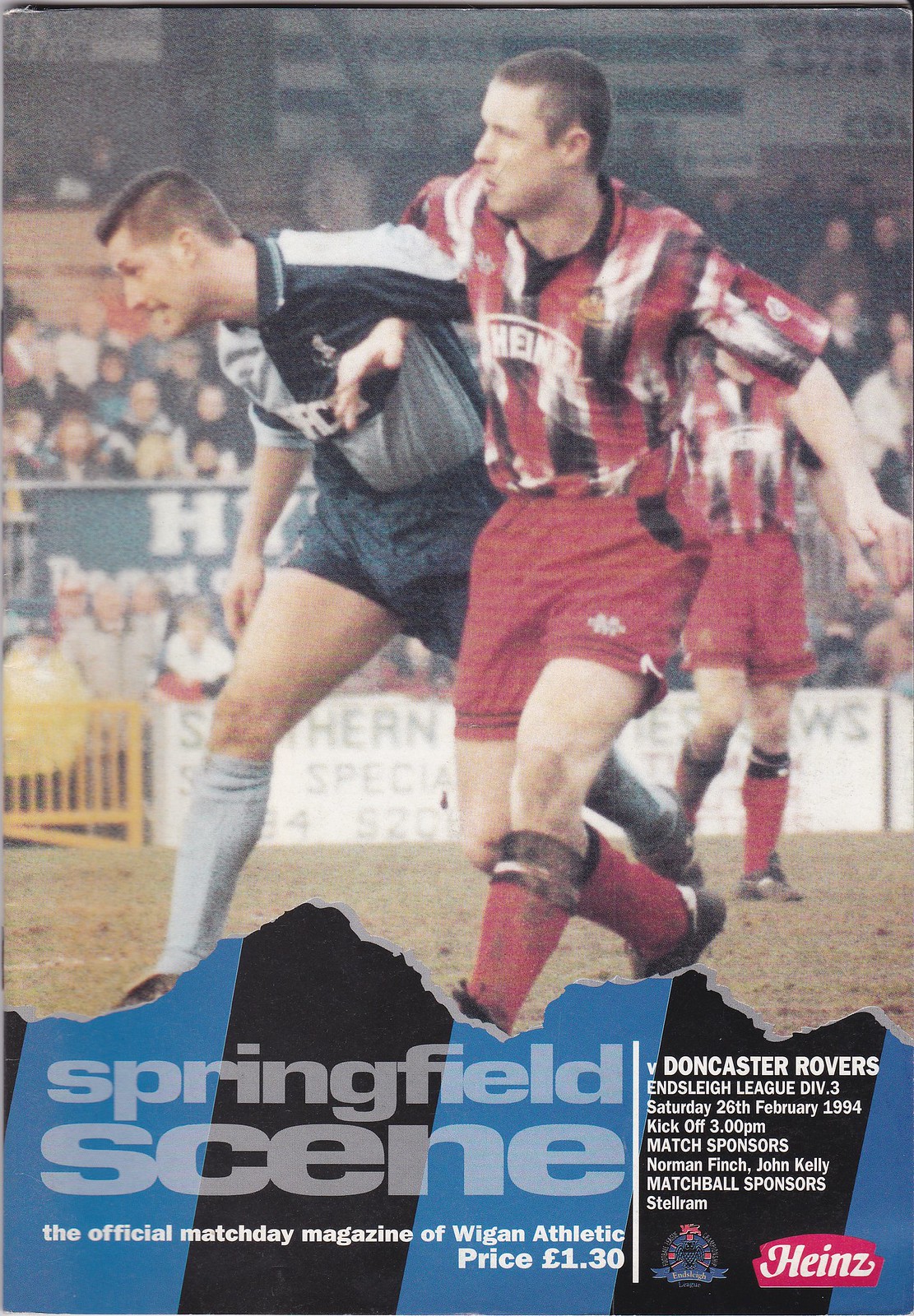The image portrays an intense soccer match scene from the front cover of "Springfield Scene," the official Match Day magazine of Wigan Athletic versus Doncaster Rovers. The foreground features two young players in a physical tussle, their arms interlocked and expressions strained as they grapple fiercely. One player is clad in a black and gray uniform with whitish-gray high-top socks, while the other is dressed in red, black, and white with matching socks. Behind them, another player's face is obscured by the foreground action, emphasizing the intensity of the encounter. The backdrop reveals a crowded stadium, full of spectators. The magazine's information is set against a striking black and blue torn-paper graphic. It details the match specifics: "Wigan Athletic vs. Doncaster Rovers," League Division III, dated 26 February 1994, with a kickoff time of 3 p.m. Sponsors and match details, including Norman Finch, John Kelly, and Stellram, are also mentioned, along with the Heinz logo at the bottom right. Priced at £1.30, this edition captures a fiercely competitive moment on the field.